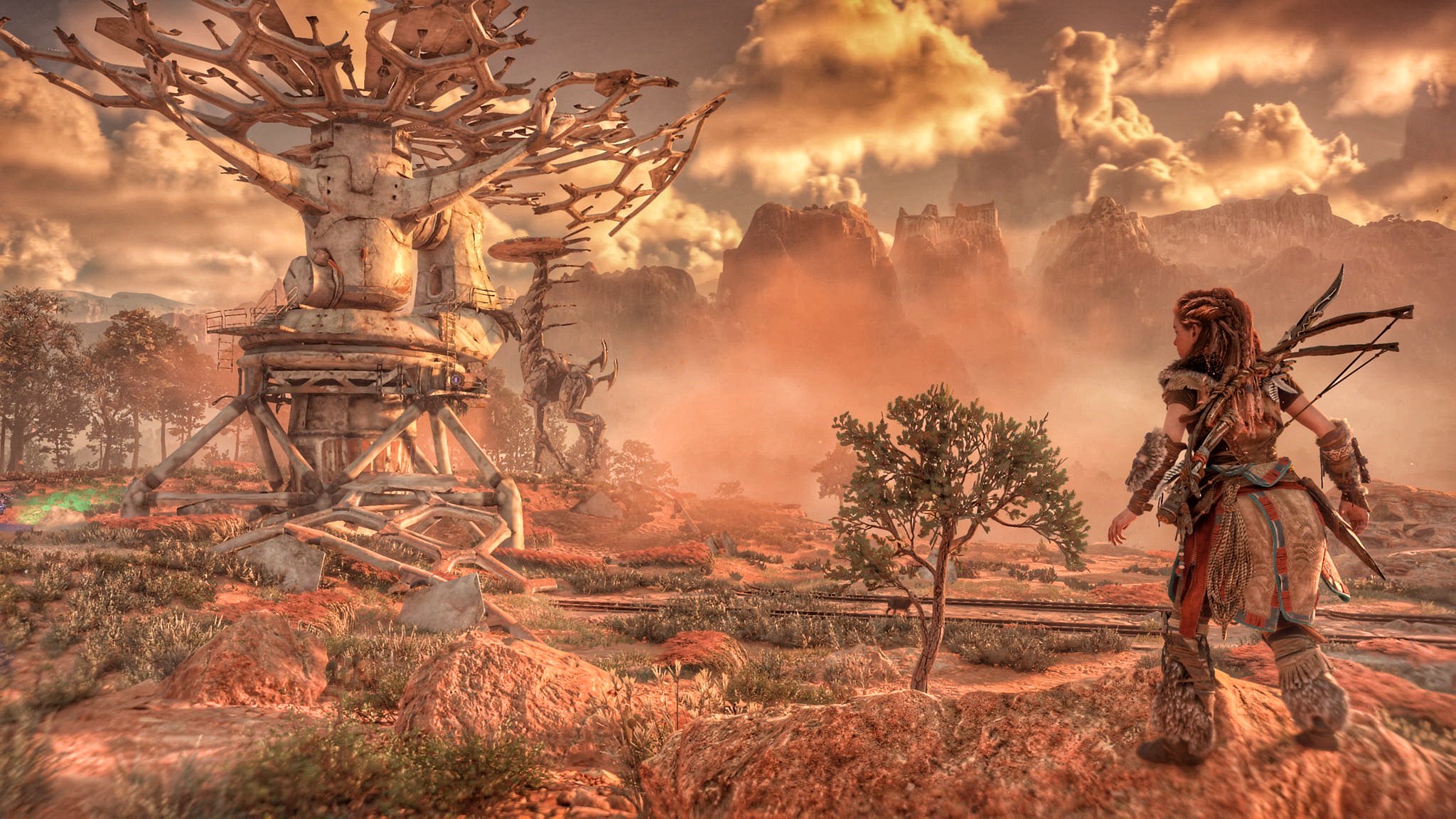In this highly detailed screenshot from a video game, the scene depicts a rough and barren landscape that evokes the vibe of an alien world or an early prehistoric civilization. The terrain is dotted with light green foliage, vast sand dunes, and mysterious pockets of mist. On the right side of the frame stands a character adorned in survivalist attire, including sheepskin and fur, with delicately braided hair. She carries two crossbows and a sword attached to her waist, suggesting she is well-prepared for any threats she might encounter. Her gaze is fixed on a treetop home or building with open gates and unconventional foundations, hinting at the unique architecture of this world. The backdrop features mist-shrouded mountains, a distant tree line, and a sky filled with scattered clouds, enhancing the enigmatic and adventurous atmosphere of the scene.